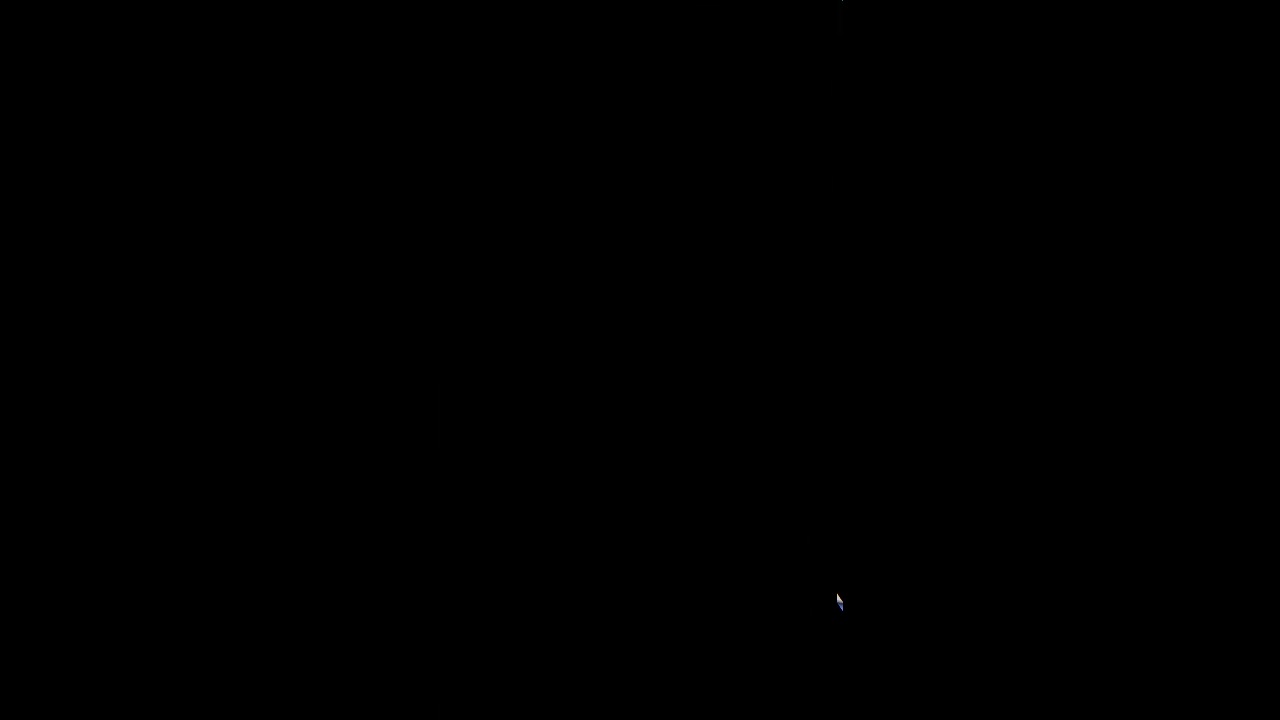This image predominantly features a uniform, pitch-black background, extending across an eight-by-four-inch landscape frame. Near the lower right corner, but slightly towards the middle, a minute kite-shaped speck can be observed—a tiny, white triangle sits atop a lighter blue triangle, reminiscent of the tip of a pen in size. This small detail stands out starkly against the otherwise pure black canvas. The image lacks any text, borders, or additional lighting, giving an impression that it might be an erroneous upload, perhaps an unsuccessful attempt at astrophotography or an accidental capture in a dimly lit room. Despite its simplicity, the image prompts curiosity due to its singular, sharply contrasting element amidst the vast black expanse.